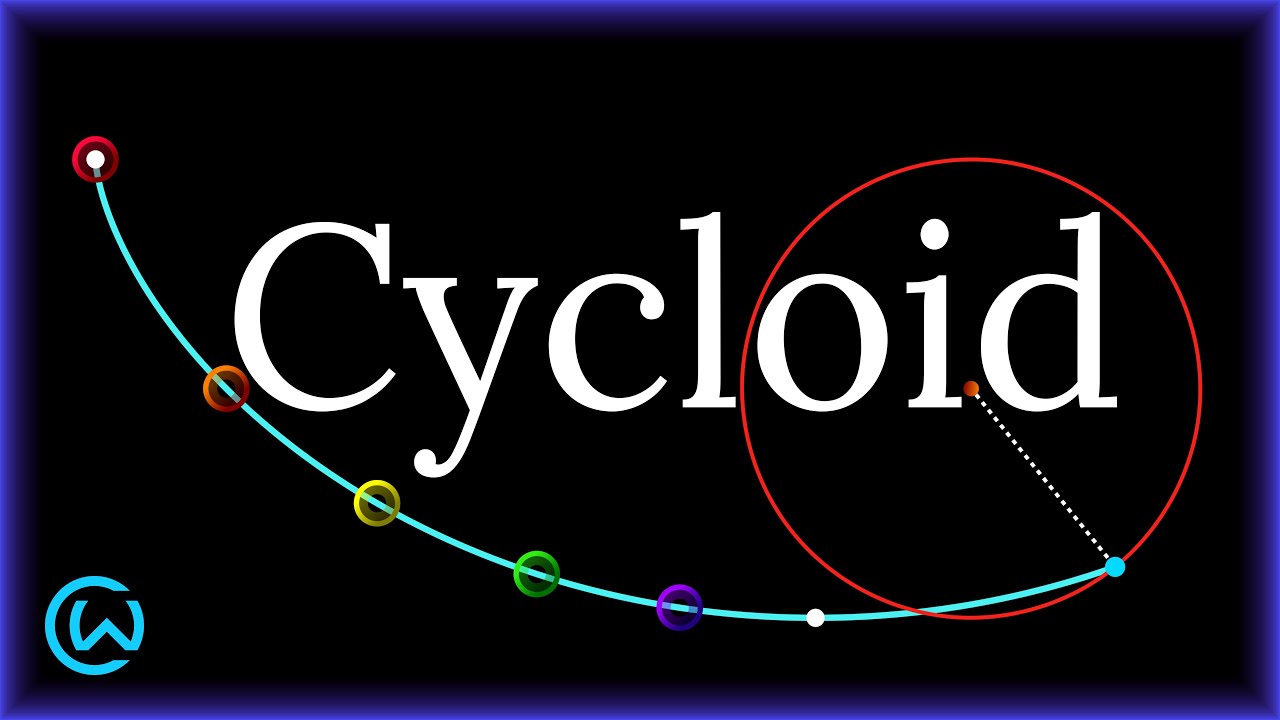The image appears to be a logo for a business named Cycloid, displayed on a rectangular, black background resembling a blackboard. The overall shape is a rectangle where the top and bottom edges are twice as long as the left and right sides. Encasing the entire image is a thin light blue border.

At the top right corner of the logo, there is a distinctive blue circle with a white "W" inside it. Prominently centered in white, bold letters is the word "Cycloid," spelled C-Y-C-L-O-I-D. 

A light blue, curved line starts near the top left corner and travels diagonally towards the bottom right before curving to the bottom left. This line intersects several multicolored circles that appear sequentially in the following order: red, orange, yellow, green, blue, white, and another blue dot. From this final blue dot, a dotted white line extends and ends in a small red dot positioned between the letters "I" and "D" in Cycloid. 

Overall, the visual elements including the multicolored circles and the curved blue line, along with the prominent "Cycloid" text, create an appealing and dynamic design, cohesively framed by the light blue border.